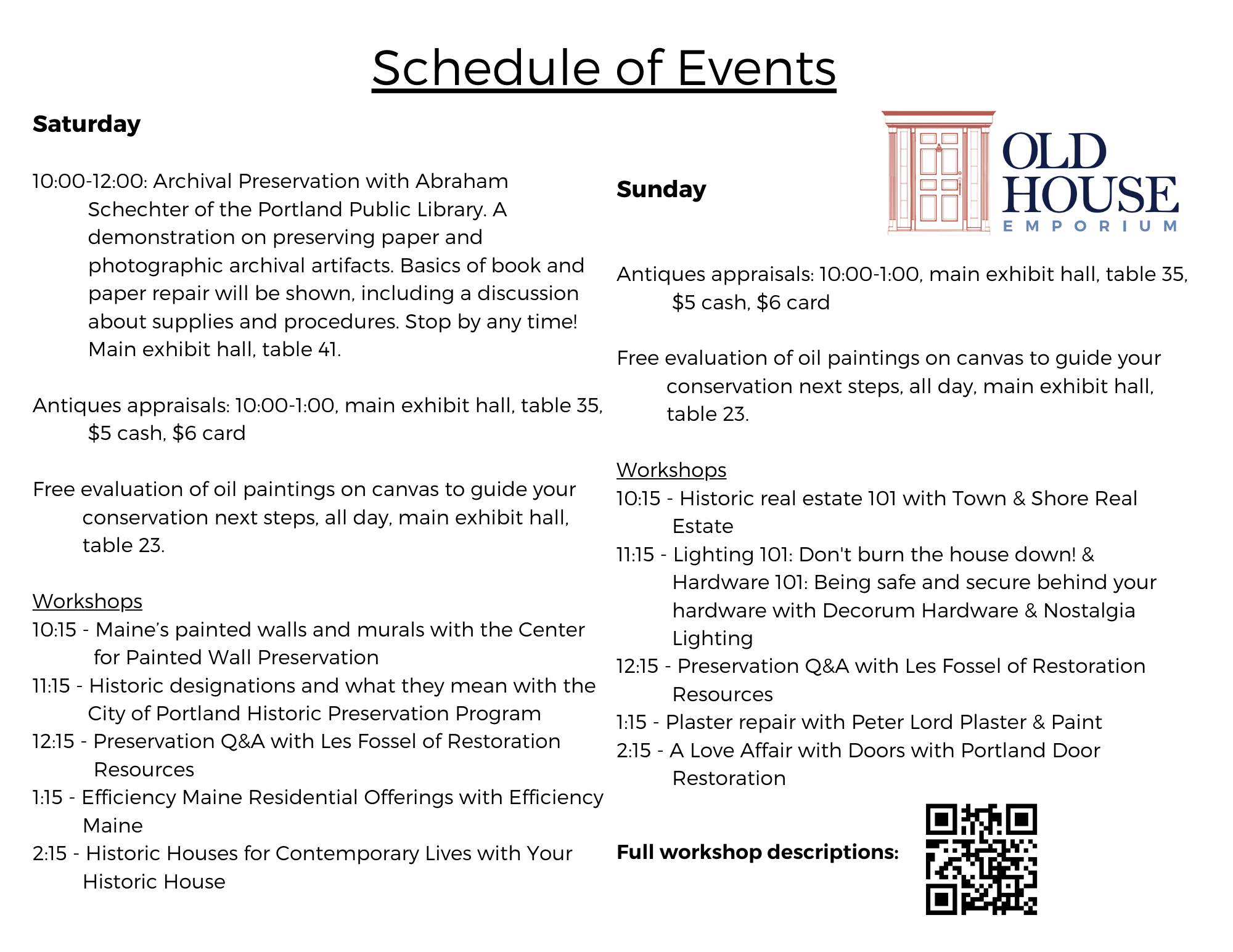This image is a detailed schedule of events for Saturday and Sunday at the Old House Emporium, featuring a door logo at the top right. The schedule outlines various activities, starting with Saturday's events, which include:

- **10:00 AM - 12:00 PM:** Archival Preservation with Abraham Schechter from the Portland Public Library. This demonstration covers preserving paper and photographic archival artifacts, and basics of book and paper repair, held at the Main Exhibit Hall, Table 41.
- **10:00 AM - 1:00 PM:** Antiques Appraisals at Main Exhibit Hall, Table 35, costing $5 cash or $6 by card.
- **All day:** Free evaluation of oil paintings on canvas to guide conservation next steps, at Main Exhibit Hall, Table 23.
- Various workshops:
  - **10:00 AM - 10:15 AM:** Maine's Painted Walls and Murals with the Center for Painted Wall Preservation.
  - **11:00 AM - 11:15 AM:** Historic Designations in Portland's Historic Preservation Program.
  - **12:00 PM - 12:15 PM:** Preservation Q&A with Les Fossel of Restoration Resources.
  - **1:00 PM - 1:15 PM:** Efficiency Maine's Residential Offerings.
  - **2:00 PM - 2:15 PM:** Historic Houses for Contemporary Lives discussion.

On Sunday, the events include similar activities:
- **10:00 AM - 1:00 PM:** Antiques Appraisals at Main Exhibit Hall, Table 35, $5 cash or $6 by card.
- **All day:** Free evaluation of oil paintings at Main Exhibit Hall, Table 23.
- Workshops starting with:
  - **10:00 AM - 10:15 AM:** Historic Real Estate 101 with Town and Shore Real Estate.
  - **11:00 AM - 11:15 AM:** Lighting and Hardware safety with Decorum Hardware and Nostalgia Lighting.
  - **12:00 PM - 12:15 PM:** Preservation Q&A with Les Fossel.
  - **1:00 PM - 1:15 PM:** Plaster Repair with Peter Lord Plaster and Paint.
  - **2:00 PM - 2:15 PM:** A Love Affair with Doors with Portland Door Restoration.

For detailed workshop descriptions, a QR code is available at the bottom right of the schedule.